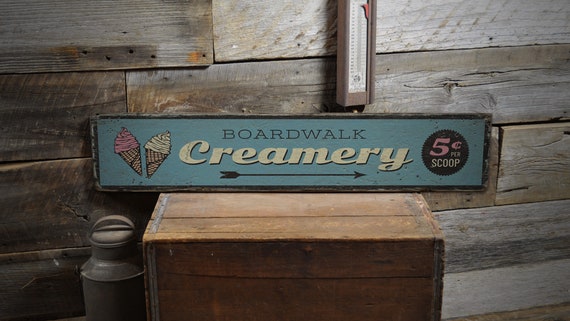The image is a horizontal, landscape-oriented close-up of a sign for a boardwalk creamery. The rectangular sign features a light blue background with two lines of text: "Boardwalk" in capitalized thin black letters at the top and "Creamery" in thick, retro white cursive at the bottom. To the left of the text, there are two waffle cones—one with pink swirled ice cream, possibly strawberry, and the other with white swirled ice cream, likely vanilla. To the right, within a small black circle, it reads "5¢ a scoop." The blue sign appears worn and is resting on a square wooden crate. Adjacent to the crate on the left is what looks like a rusted milk can or a similar jug. The entire setup is positioned in front of a wall made of wooden planks. Above and to the right on the wall, there is a thermometer or some type of measuring device, adding to the rustic feel of the scene. The setting is well-lit, highlighting the details of the objects and their textures.